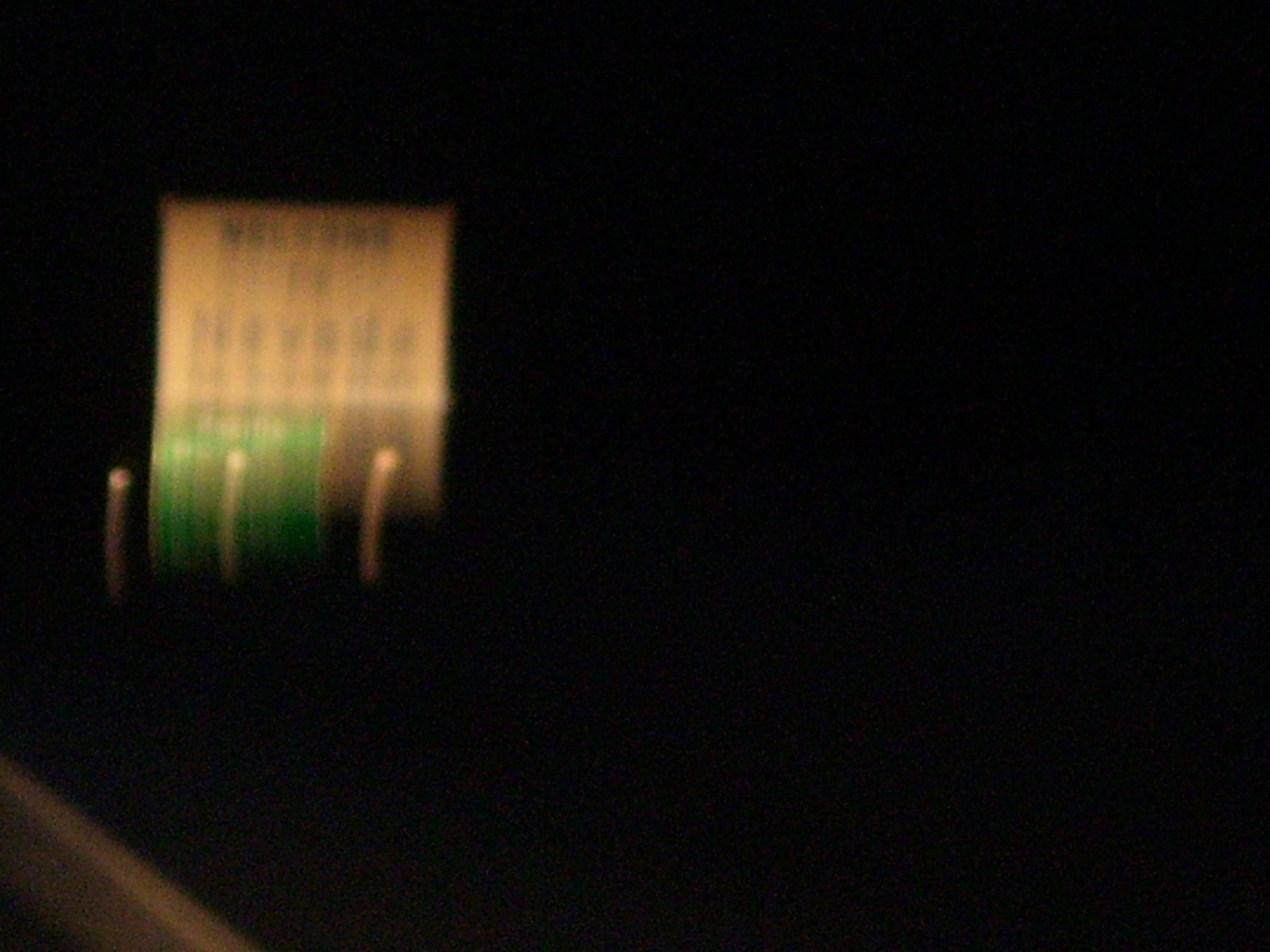This is a nighttime photograph captured from a moving car, resulting in a very blurry image. The darkness and motion make it challenging to discern details, but the focal point appears to be a white rectangular sign with blue letters and a blue border, which likely reads "Welcome to Nevada." This sign is elevated, possibly on a pole. Below it, to the left, there seems to be a green square sign that resembles a street sign, indicating highway information. The photo also shows three blurred beams of light near the bottom, possibly from the car’s headlights, and a small visible stretch of road in the bottom left corner. Additionally, part of a car window trim, which appears gray, is slightly visible in the frame, indicating the photo was taken from inside the vehicle.